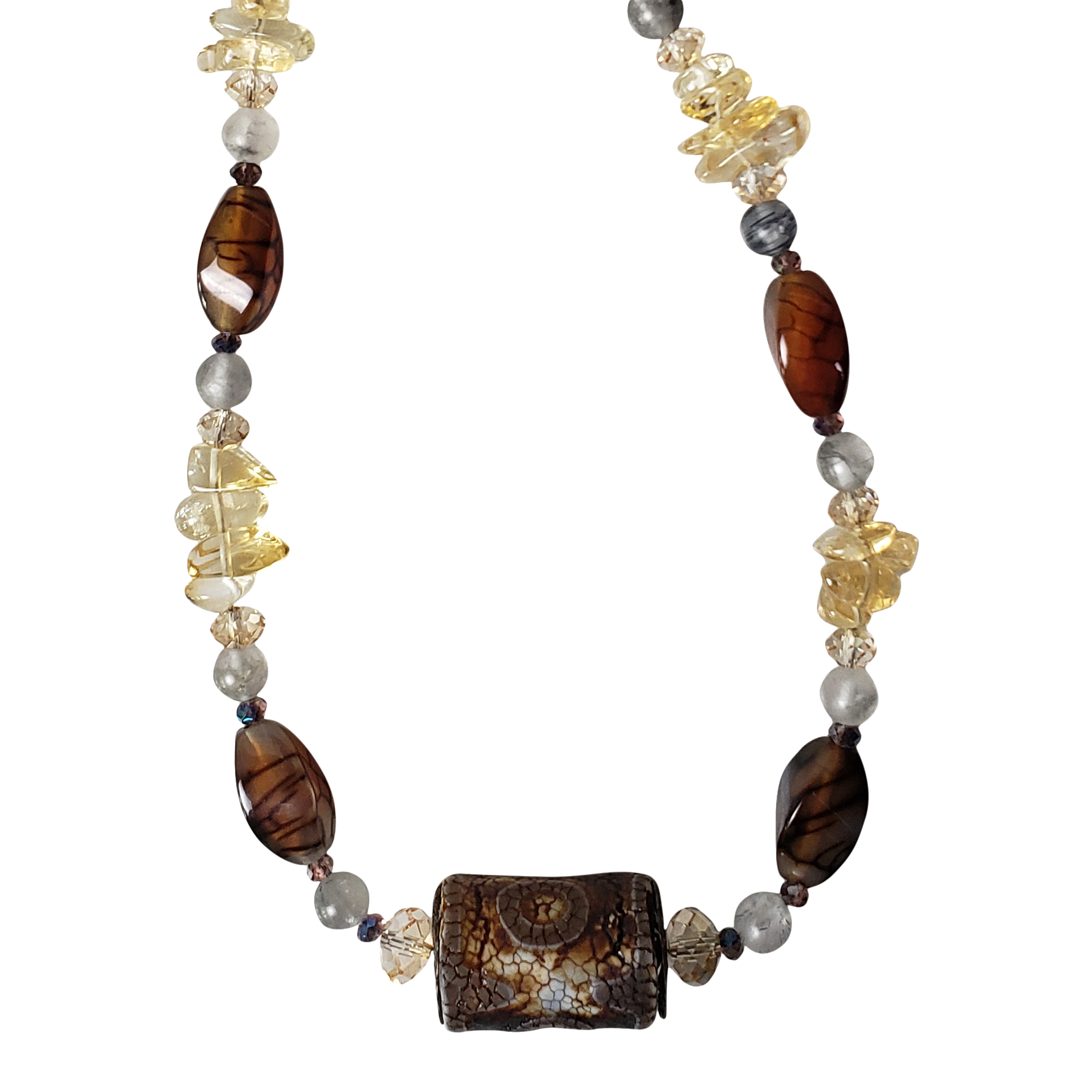The close-up image captures a necklace intricately composed of various gemstones against a stark white background. The necklace strand begins on the right, descends to the bottom of the frame, and arcs back up to the left without showing the clasp. The stones and beads adorning the necklace range in shape, size, and color, tightly clustered together in an alternating pattern. Notable features include steel-gray beads, cream-colored stones with rough edges, a transparent brownish oval stone embedded with rocks, and a distinctive, larger oval stone with gray and black streaks. At the strand's lowest point, a cylindrical bead is prominently featured, showcasing a dry, cracked pattern in hues of white, brown, cream, and gold. The left side mirrors the right with a symmetrical arrangement of the same diverse elements. The image is set in bright, natural light, highlighting the clear details and the varied textures of the gemstones, producing a vivid and detailed visual representation.